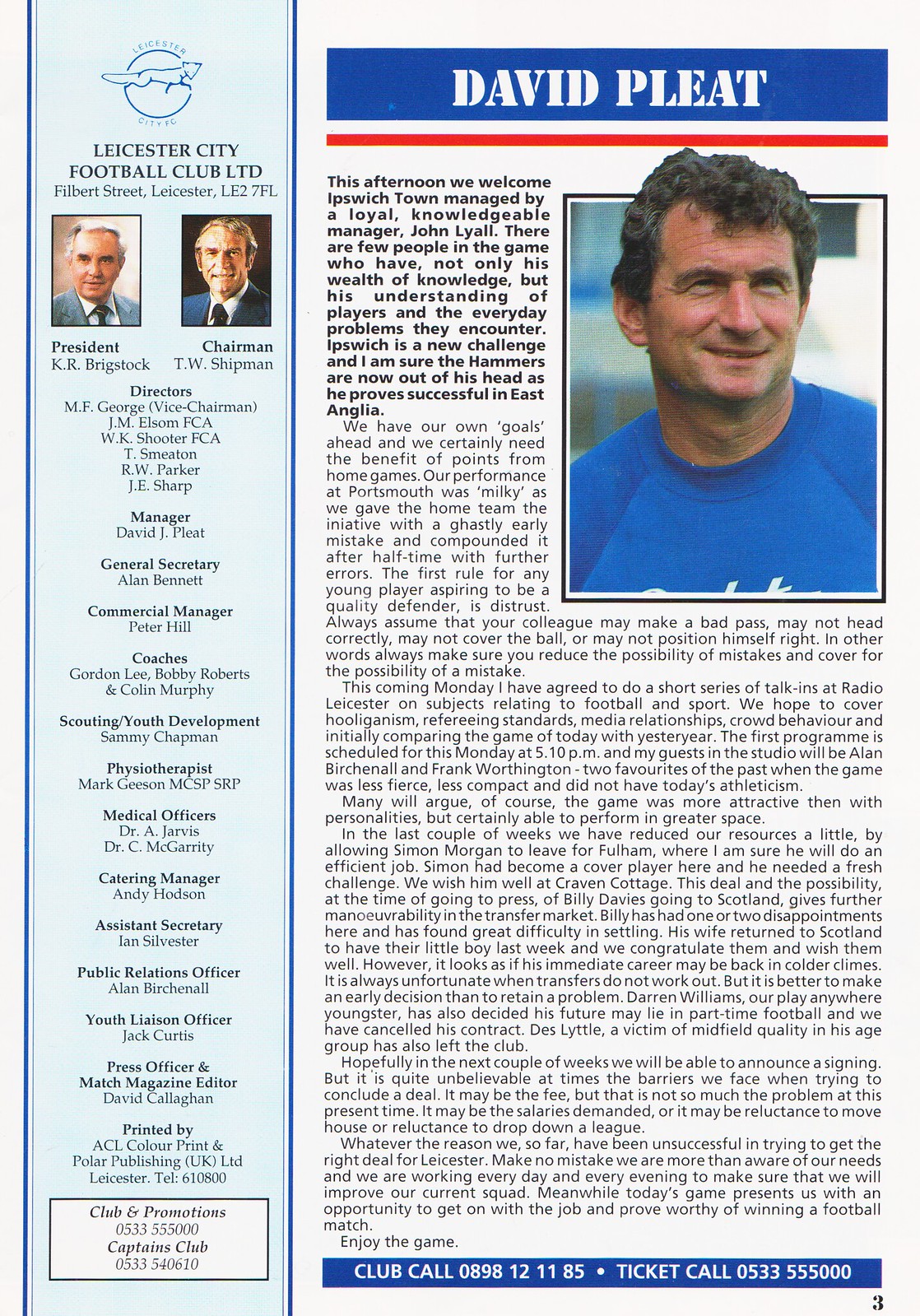This image is a detailed photograph of a page taken from what appears to be a British football club magazine, specifically Leicester City Football Club Limited. Dominating the left side of the page is a light blue strip with a fox logo at the top, labeled "Leicester City Football Club Ltd, Filbert Street, Leicester, LE27F1." This section includes headshots and titles of key personnel like President K.R. Brigstocke and Chairman T.W. Shipman, followed by a comprehensive list of directors, managers, officials, and their respective titles. It ends with multiple contact numbers for club services and ticket inquiries.

On the right side, taking up two-thirds of the page, is a column authored by David Pleat. The header of this section features Pleat's name in bold white letters on a blue background, bordered beneath by a thin red line. Just below the header is a headshot of David Pleat, a Caucasian man in his late 30s to early 40s with light brown curly hair, smiling and dressed in a blue shirt. The column starts with a welcome note to Ipswich Town, discussing its manager John Lyle's expertise and experiences, and further elaborates on team goals and challenges in several paragraphs. Near the bottom, in a blue strip with white font, the page lists additional phone numbers for club and promotional inquiries as well as ticket information.